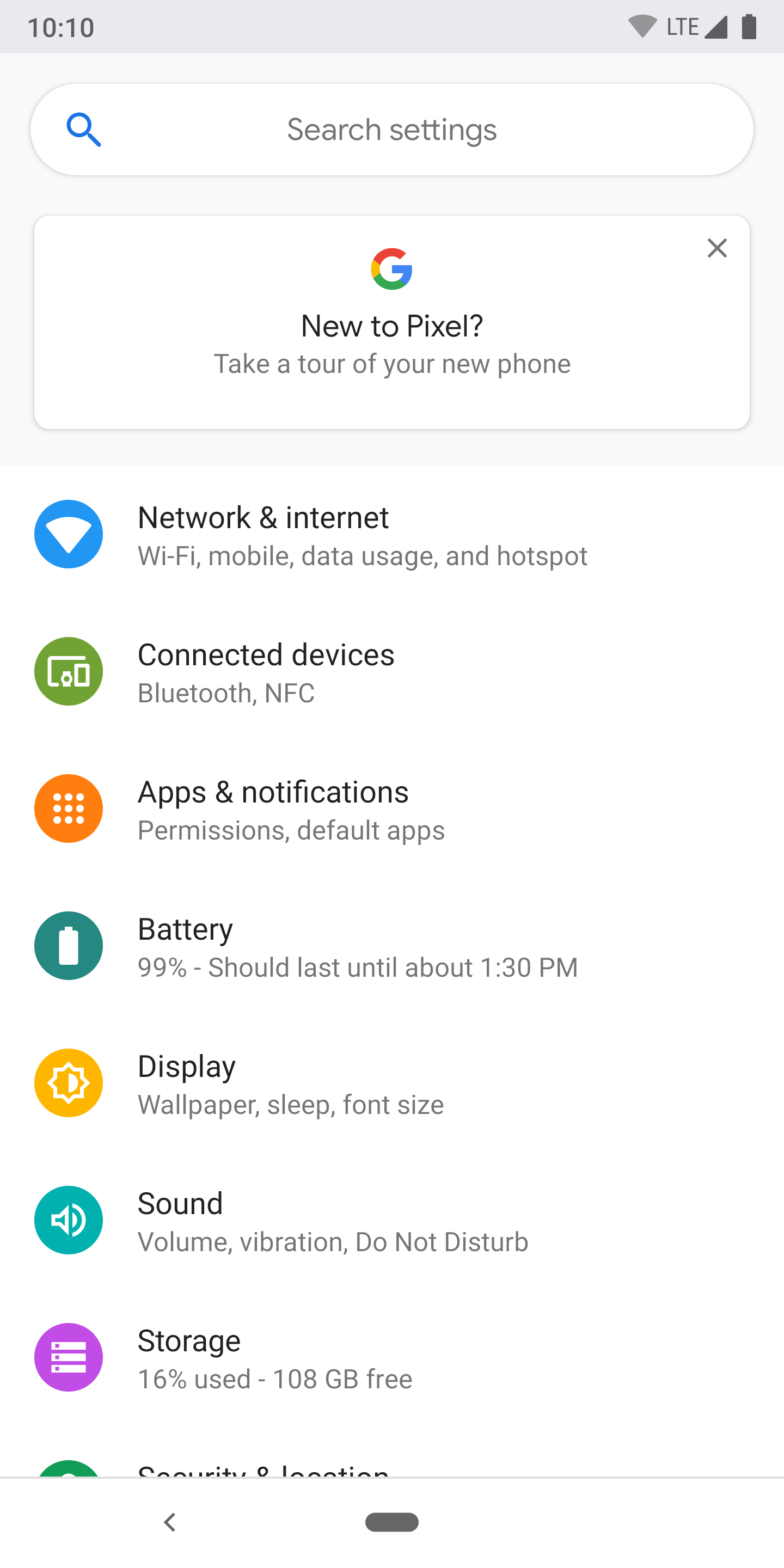Screenshot of the Settings page on a Google Pixel phone. The time displayed at the top is 10:10, accompanied by status icons on the right indicating Wi-Fi connectivity, mobile data, and battery level. Beneath the status bar is a search option labeled "Search settings." Below the search bar, there is a pop-up window featuring the Google icon with the message "New to Pixel? Take a tour of your new phone," and an "X" in the upper-right corner to close the pop-up.

The main Settings menu is listed with its corresponding icons in various colors. The items in the menu, from top to bottom, include:
1. Network & Internet 
2. Connected devices 
3. Apps & notifications 
4. Battery 
5. Display 
6. Sound 
7. Storage

Each icon is distinctly colored and appropriate to its respective setting category. The colors of the icons include blue, olive, dark orange, teal, light orange, light teal, and purple. The background of the Settings page is white, with black text for the menu items.